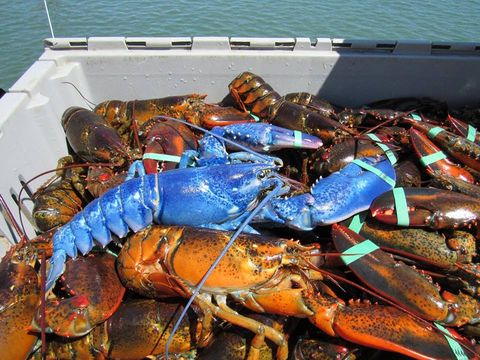In this outdoor photograph likely taken on a vessel, we see a grayish-white plastic container floating in blue, rippling ocean water. The container, which has strings on its sides to hold it up, is filled with dozens of lobsters. All the lobsters, sporting long antennae and claws bound with green rubber bands, are closely packed atop one another. The majority of them are the typical reddish-orange color with black or brown spots. However, prominently placed on top of the pile is a striking blue lobster with white tints and fringes, making it the focal point of the image. This unique blue lobster is facing right, with one fully black eye visible. The open lid of the container and the shadow across its right side suggest that this image was captured during a bright, sunny day as part of a successful crab and lobster-catching expedition.